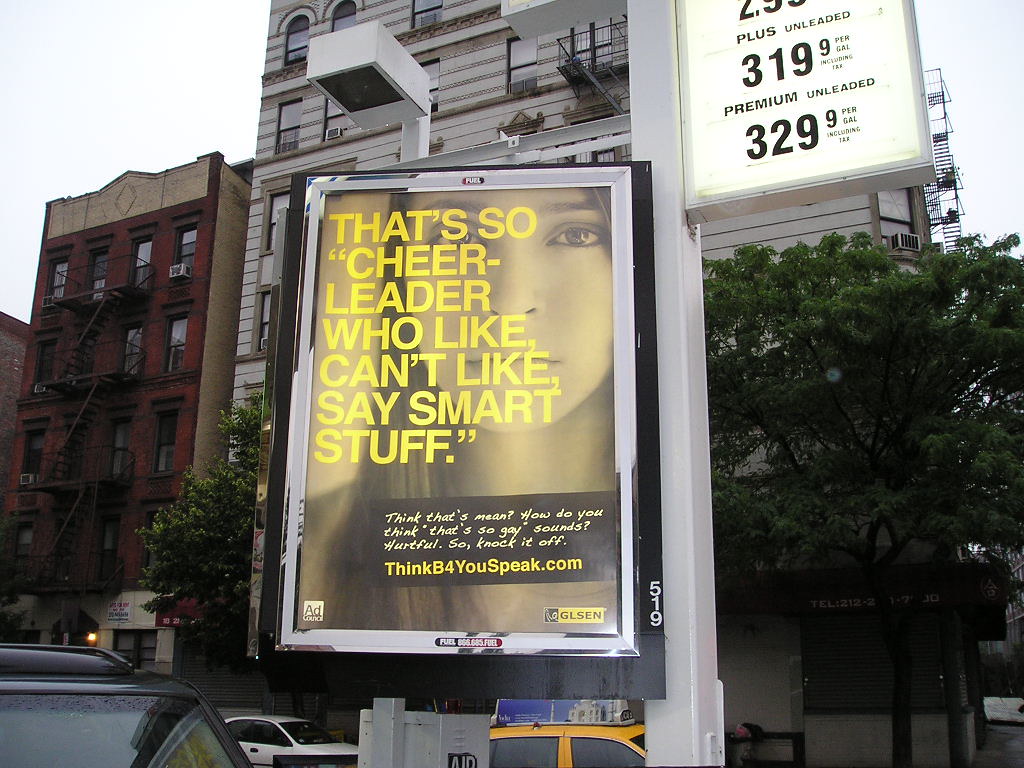In this cityscape photograph, a prominent tall building stands in the background, creating an urban atmosphere. Dominating the foreground is a silver-framed billboard attached to a post, featuring a notable advertisement for thinkbeforeyouspeak.com. The ad showcases a girl's face as the background image with a bold, yellow text that reads, "That's so cheerleader who like can't like say smart stuff," highlighting its message. Below the billboard, a few cars are parked on the street, adding to the bustling city setting. To the left of the billboard, there is a red brick building, while to the right, the scene includes some leafy trees and a sign displaying current gasoline prices.